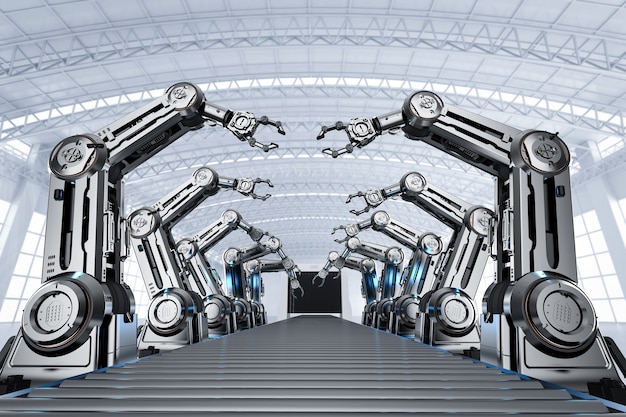The image depicts an assembly line in what appears to be a factory or hangar, featuring a prominent black conveyor belt flanked by ten large, silver-gray, metallic robotic arms—five on each side. The robotic arms are positioned upright, seemingly poised for action, and appear capable of extensive mobility, including vertical and horizontal movements. The background of the image is predominantly white and gray with muted tones throughout, suggesting an industrial environment. Large windows on the left and right sides allow natural light to flood the space, highlighting the intricate crisscross girders supporting the high ceiling. The scene exudes a high-tech ambiance, potentially part of a robotics facility, and the overall aesthetic hints at a stylized illustration, possibly resembling a comic book or AI-generated art.